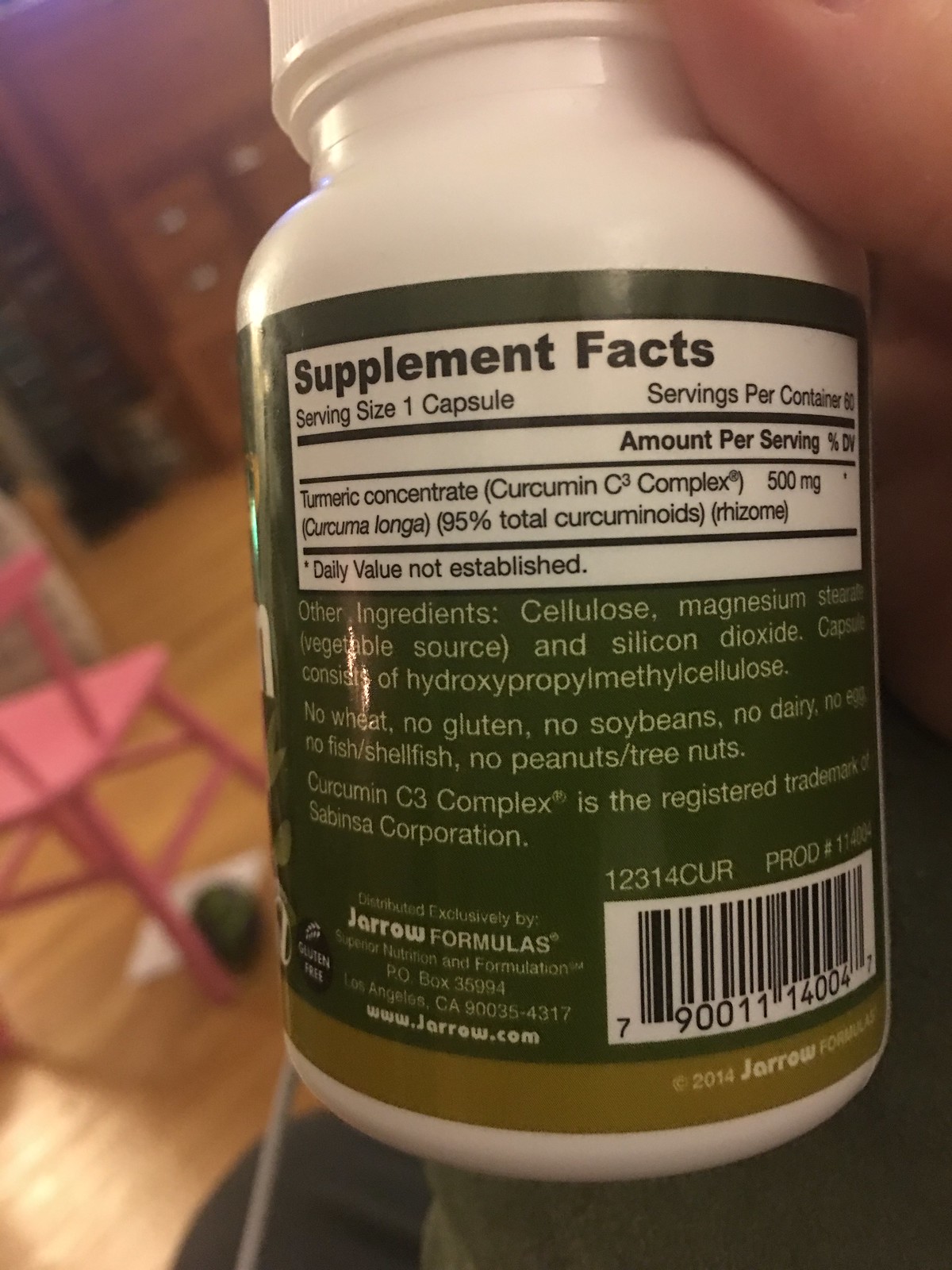A detailed, descriptive caption for the provided image could be:

"This photograph features a white bottle of turmeric caplets, specifically capturing the back label that details the supplemental facts. The label, dominated by a green background with white text, enumerates the contents, revealing a serving size with 500 mg of turmeric concentrate. On the lower right corner of the bottle, a barcode is present, while the brand name 'Jarrow Formulas' is printed to the left of the barcode. The backdrop of the image offers a glimpse into a cozy living space or office, showcasing a pink chair, a set of drawers, and a light wooden floor, enriching the context of the scene."